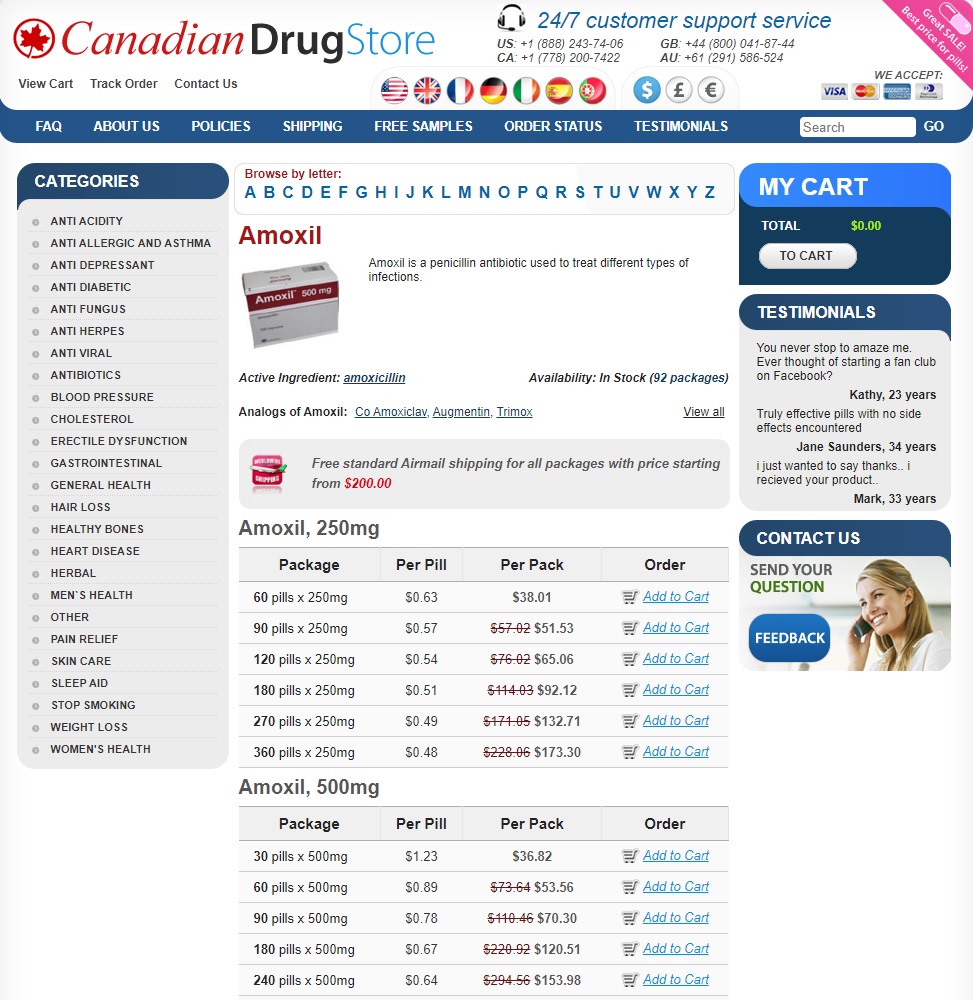The image is a screenshot of the homepage of a company website called "Canadian Drugstore." The header of the page is a light blue color, prominently featuring a Canadian maple leaf icon in a red circle. To the right of the icon, the word "Canadian" is written in red text, "Drug" is in bold black text, and "store" is in blue text. In the upper right corner, the text "24-7 customer support service" is displayed.

Beneath the header, there is a dark blue banner with a horizontal menu in white text, listing the following options from left to right: "FAQ," "About Us," "Policies," "Shipping," "Free Samples," "Order Status," "Testimonials," and a white search bar at the far right end of the menu.

On the left side of the webpage, there is a sidebar titled "Categories," listing various product categories in vertical arrangement. These categories include: "Anti-Acidity," "Anti-Allergic and Asthma," "Anti-Depressant," "Anti-Diabetic," "Anti-Fungus," and "Anti-Herpes."